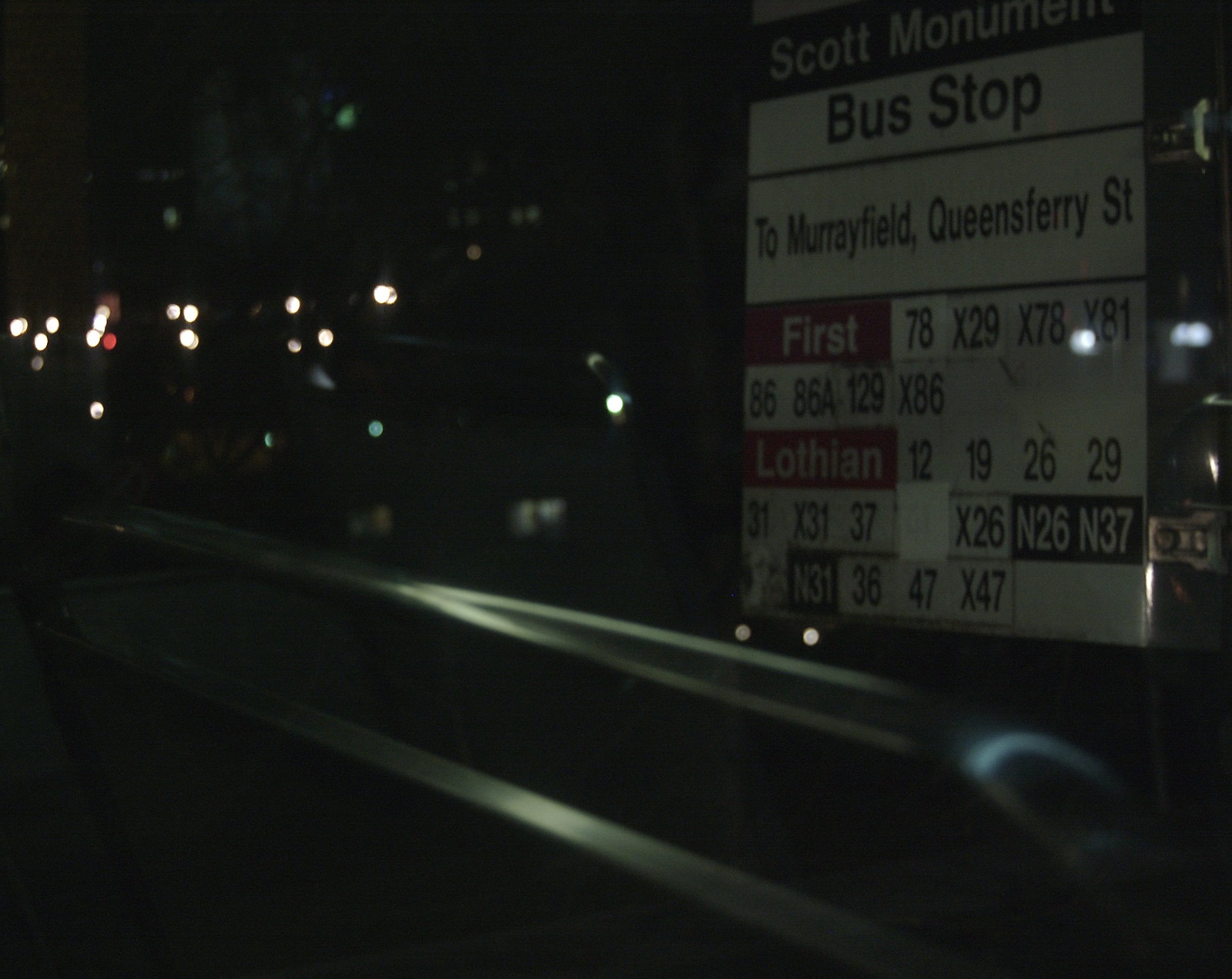In this nighttime photograph, the viewer's perspective is angled toward a bus stop sign. A railing or banister is in the foreground, and there's a subtle reflection suggesting a glass surface. On the sign, at the top, "Scott" and "M-O-N" are visible, followed by "bus stop." Below, in clearer text, it lists destinations: "to Murrayfield, Queensferry Street." Various route numbers and letters are displayed on banners, including "78, X29, X78, X81," "86, 86A, 129, X86," and "12, 19, 26, 29." Additional routes in smaller text include "31, X31, 37, X26, N26, N37, N31, 36, 47, X47." To the right, more numbers such as "12, 19, 26, 29" are repeated, framed by the names "First" and "Lothian." The scene is illuminated by city lights beyond the sign, casting reflections and creating a chiaroscuro effect against the otherwise dark environment.